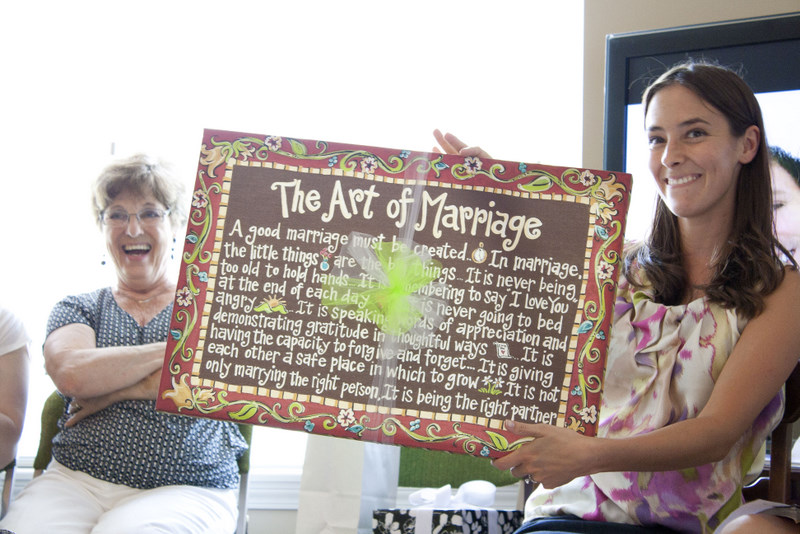The image depicts a young woman and an older woman smiling together, both of them seated. The young woman, who has brown hair that is wavy at the ends and falls just past her shoulders, is holding a rectangular sign with a floral border embellished in gold and blue flowers and leaves. The sign prominently reads "The Art of Marriage" in white letters, though the rest of the text is hard to decipher due to a white and yellow color obstruction, possibly from paint or lighting. This sign also contains more text about marriage, beginning with "A good marriage must be created" and mentioning that "the little things are the best things," followed by several other lines. 

The older woman, Julia, is smiling broadly, with her blonde hair cut short, and she’s wearing glasses. She is dressed in a short-sleeved polka dot blouse and white shorts, with her arms crossed at her chest and partially covered by the sign. The background is a bright, whitewashed space, suggesting a cheerful, well-lit indoor setting, potentially at a party or get-together celebrating the theme of the sign. The atmosphere captured in the image portrays a moment of joy and warmth shared between the two women.